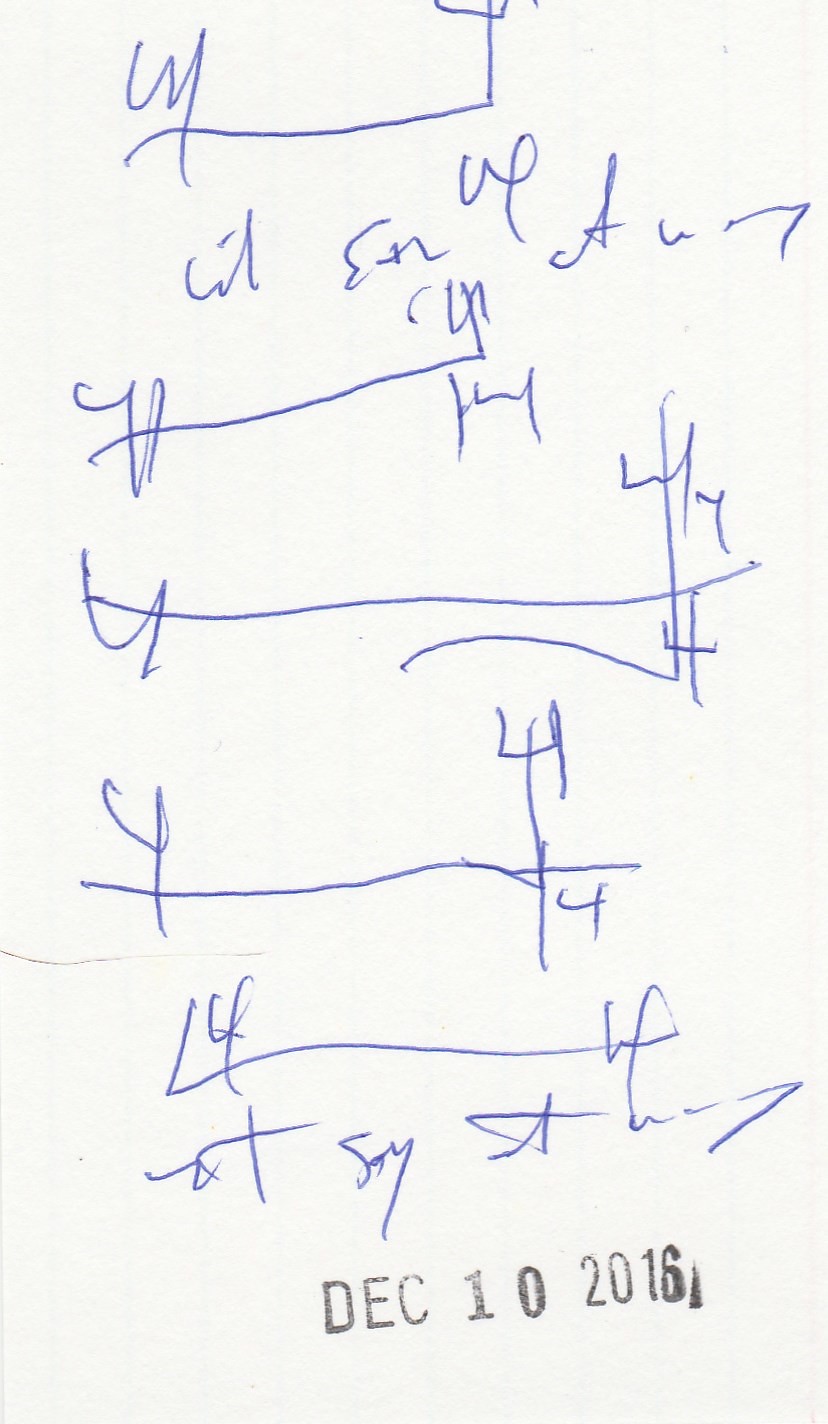The photograph captures an entire piece of white paper, filled with blue biro scribbles. Dominating the page are a multitude of intersecting lines, many forming the shapes of the letter 'Y' and the number '4,' though some might resemble intersections or trident figures. The overall arrangement of these lines suggests a form of gameplay or coded message, meaningful to the intended recipient. Towards the bottom edge of the paper, a date stamp in black ink reads "December 10, 2016." Aside from this, there are two lines of completely illegible scribbled text. The background provides no additional context as only the paper itself is visible.